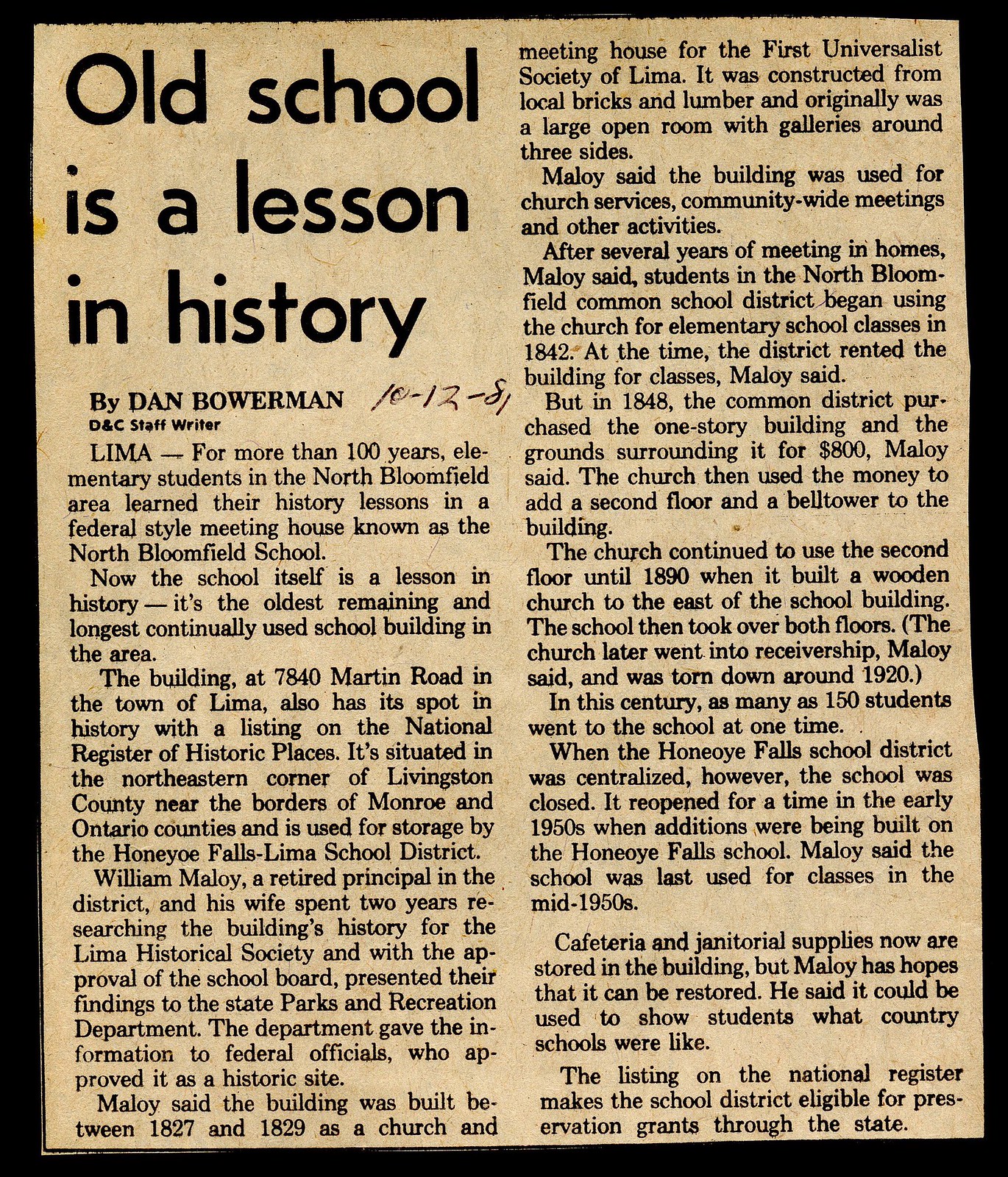This image features a color photograph of an old, yellowed newspaper clipping with black print. The top left corner of the clipping displays a bold title that reads, "Old School is a Lesson in History." Directly below the title is a byline in slightly smaller text, attributed to Dan Bowerman, DNC Staff Writer. A handwritten date, "10-12-81," appears to the right of the byline. The article begins with the word "Lima" in large type, indicating the location, and proceeds to describe how, for over 100 years, elementary students in the North Bloomfield area learned their history lessons in a federal-style meeting house known as the North Bloomfield School. The text is arranged in multiple paragraphs, split into two columns and set against a black background, suggesting the clipping might have been scanned.